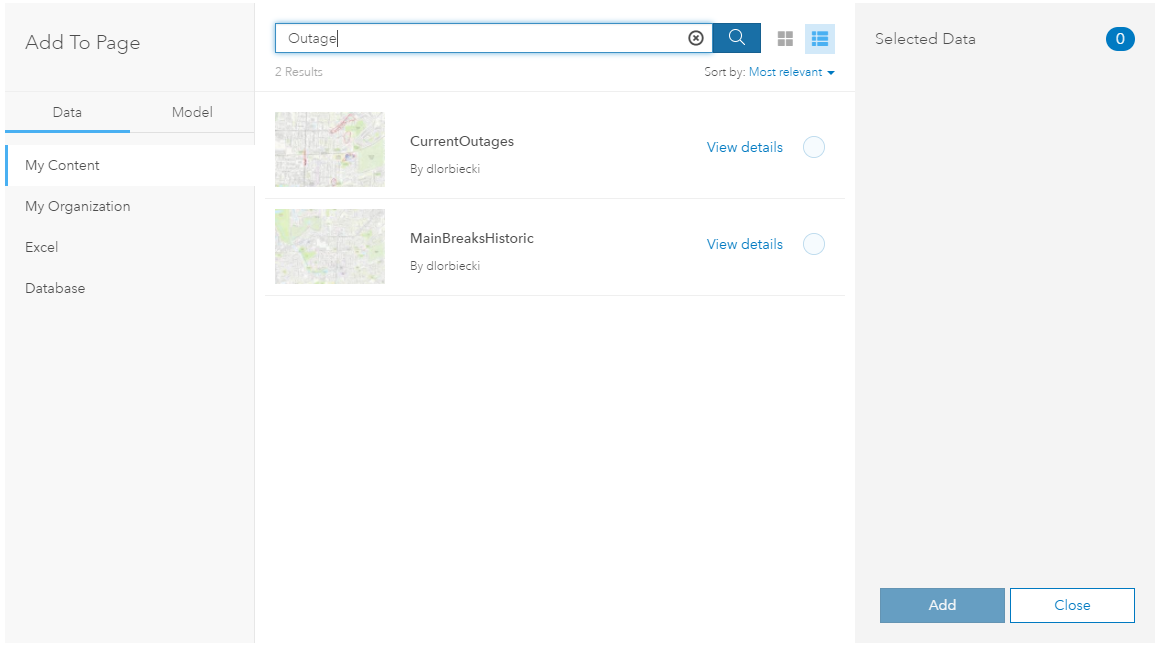The image displays a web page in landscape orientation designed for searching and viewing information about outages. The webpage is divided into three main sections:

1. **Left Sidebar (Light Gray Column)**: This column is titled "Add to Page." Beneath the title, there are two tabs labeled "Data" and "Model," with "Data" currently selected, indicated by a blue underline. Under the "Data" tab, there are four categories listed: "My Content," "My Organization," "Excel," and "Database." The category "My Content" is highlighted, marked by a white rectangular background and a vertical blue bar on its left side.

2. **Center Section (White Background)**: The main part of the page features a search bar at the top, outlined in blue. Inside the search bar, the word "outage" has been typed. To the right of the search bar, there is a circle with an X, presumably for clearing the input. Adjacent to this is a dark blue square containing a white magnifying glass icon, used to initiate the search. Below the search bar, the page displays "True Results" followed by "Sort By," which is currently set to "Most Relevant." This can be changed via an arrow icon next to it. The search results include thumbnails of maps. The first result is titled "Current Outages" by an author whose name appears to be "Dior Biecki." To the right of this title is a clickable "View Details" blue link. The second result is another map labeled "Main Breaks Historic," also by "Dior Biecki," with a similar "View Details" link. The remainder of the center section is blank.

3. **Right Sidebar (Light Gray Column)**: This column is titled "Selected Data," with a blue oval containing an "O." The rest of this column is blank until the bottom, where two buttons are located: "Add," which is a blue rectangle with white text, and "Close," a white rectangle with blue text and a blue outline.

Overall, the layout is user-friendly, allowing easy navigation and operation for searching and managing data related to outages.